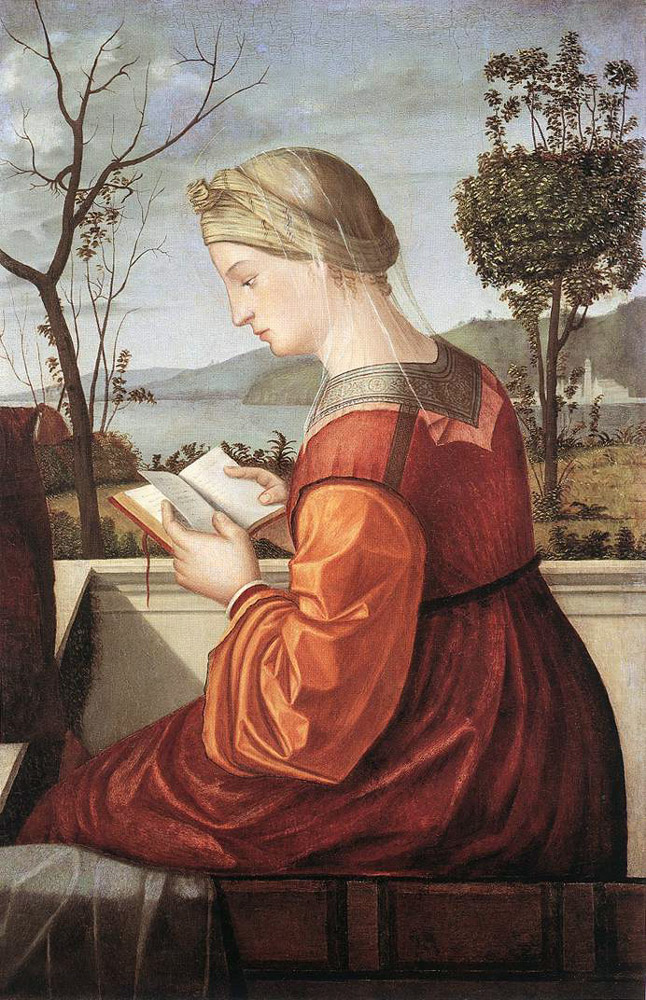The painting depicts a young woman seated on a brown wooden bench, engrossed in reading a small book with a red cover, which she holds open at chest level. She wears a red dress with orange sleeves and a distinctive metallic bronze neckline that tapers to a point near her shoulder blades. Her head is adorned with a light brown scarf and a see-through net-like veil that drapes over the back of her neck. The woman's alabaster skin contrasts with her brightly colored attire. Her right index finger holds down the book's open pages, while her left finger is poised under one of them, suggesting she is about to turn the page. 

Set in an outdoor scene, a white barrier is visibly positioned in front and behind her. To her right, a lush tree with dense foliage reaches upward, while to her left, a dead tree with sparse, withered branches stands in stark contrast. The background reveals a serene body of water, with the landscape transitioning to distant mountains under a brooding, purple-gray sky that hints at impending rain. The overall ambiance, along with the flat, non-dimensional style of the painting, suggests it could be from the 14th or 15th century, exuding an old-fashioned charm.